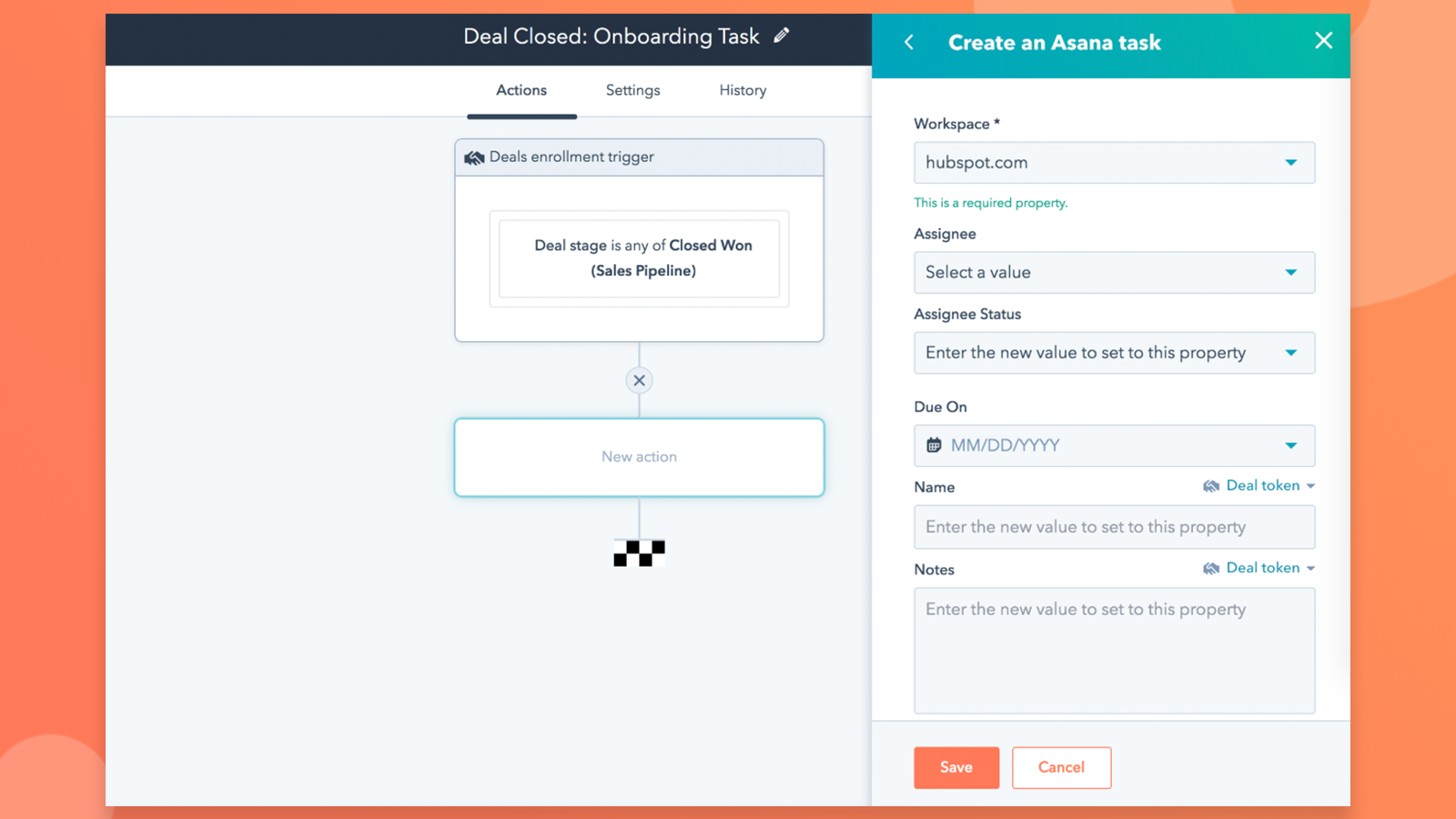Screenshot description: 

The screenshot features a user interface bordered with an orange frame. At the top, a black rectangle contains the text "Deal Closed Onboarding Task." Below this, the background turns white with black text displaying three options: "Actions," "Settings," and "History." 

Under these options, the phrase "Deals Enrollment Trigger" is prominently displayed, followed by a box outlining the criteria: "Deal stage is any of 'closed won' (Sales Pipeline)." 

A line emerges from this box, connecting to another box outlined in turquoise labeled "New Action." Further to the right, the interface indicates the option to "Create Asana Task," linked to a workspace identified as "hubspot.com" (a required property).

Several fields are available for user input:
- **Assignee:** A dropdown to select a value.
- **Assignee Status:** A field to enter a new value for the property.
- **Due on:** A date selection box.
- **Name:** A field to input a new value for the property.
- **Notes:** An area to take additional notes.

At the bottom, two buttons are visible: an orange "Save" button and a white "Cancel" button with an orange border. This concludes the elements displayed in the screenshot.